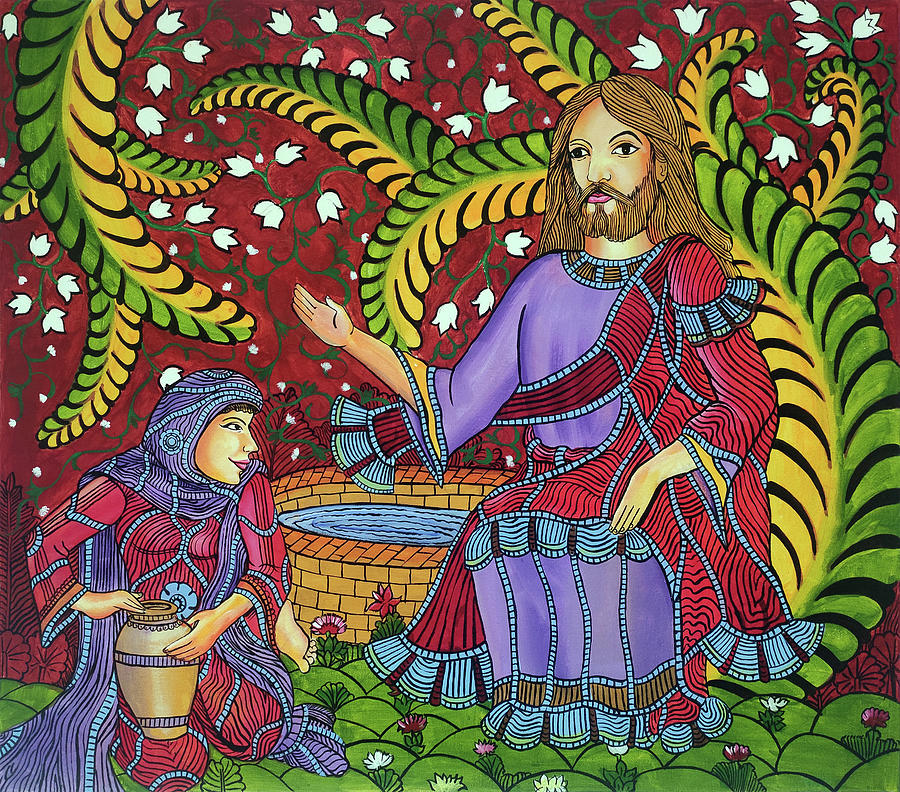The image is a colored drawing in a large square format, depicting a scene involving two primary figures against a vibrant background. The central figure is Jesus, identifiable by his serene expression, long brown hair, and brown beard. He is adorned in a purple robe featuring an intricate, beaded red shawl with black wavy lines. Jesus extends his right palm outward, towards the viewer's left. 

To the bottom left of Jesus, there is a kneeling woman. She is dressed in a red-colored dress with a blue-purple beaded hood that flows down her neck and acts as a cape. The woman, smiling, holds a golden-colored urn with both hands, resting it on her right knee. The ground where she kneels is green, adorned with small flowers.

In the background, a circular brick-bordered pond with water is visible beside the kneeling woman. The backdrop features a rich red hue with large, curved green and yellow leaves and thin green stems adorned with white flowers, creating a lush, captivating environment.